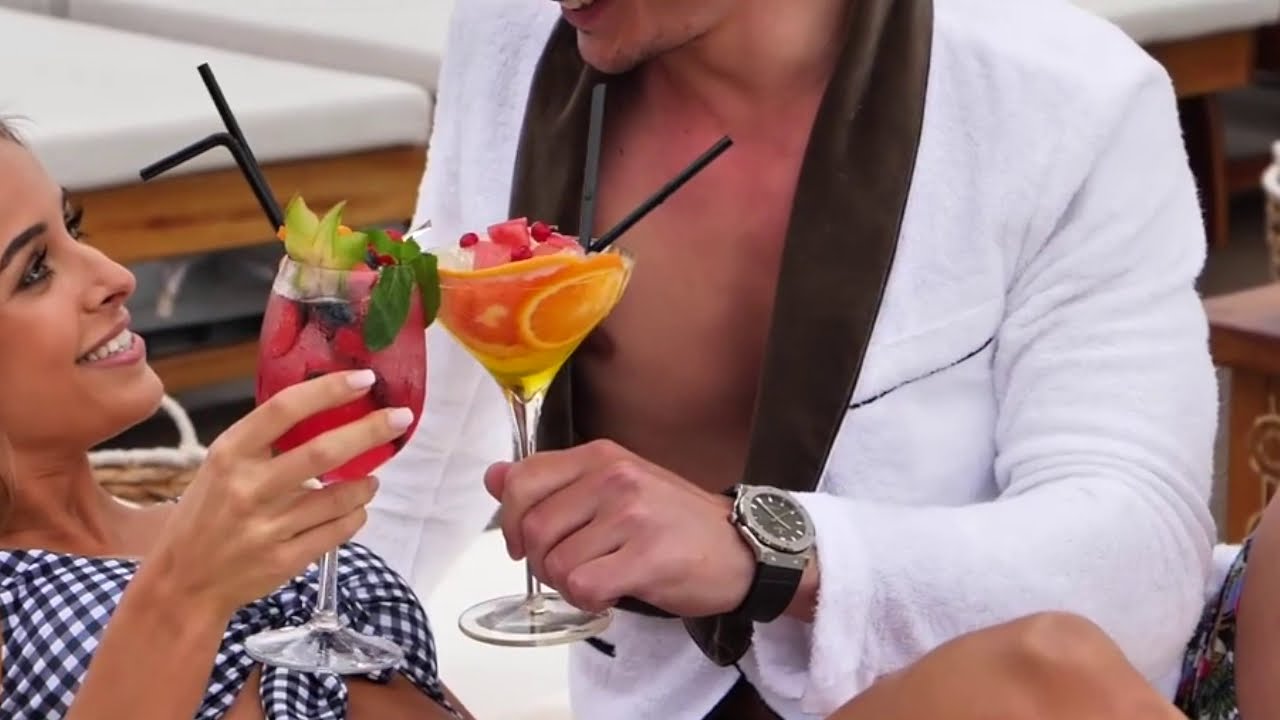The image is a close-up of a smiling woman and a man toasting with cocktails, likely on a beach vacation or at a luxurious hotel. The woman's face is fully visible, showing her makeup and lipstick. She is lying back on a beach chair with white padding, wearing a black and white checkered bathing suit top tied at the center. In her right hand, she holds a red cocktail garnished with an assortment of fruit and mint, along with two black straws. The man sits beside her, his face mostly out of frame, visible only up to his chin. He is shirtless but wearing a white robe with brown collars and a stylish watch on his left wrist. He holds a martini-style glass containing a light yellow-orange drink decorated with fruit, including oranges, melons, and berries, also with two black straws. Behind them, wooden paneling with white accents can be seen, suggesting a boat or a similarly adorned area.